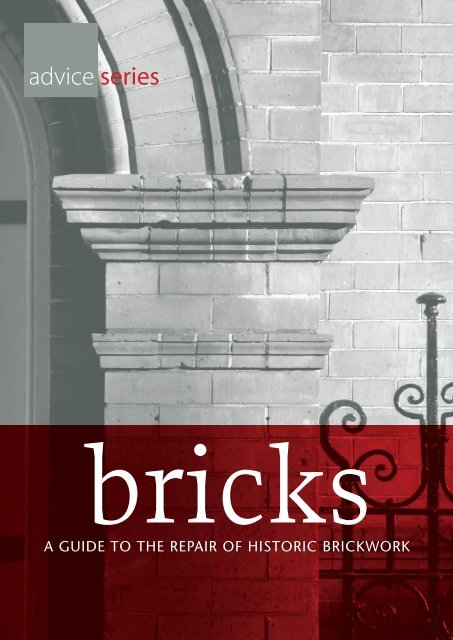This image appears to be the cover of a guide or brochure, featuring a detailed black and white photograph of a historic brick archway seamlessly incorporated into a brick wall backdrop. On the top left, overlaid in a gray box, the word "Advice" is prominently displayed in white, followed by "Series" in a striking red color. To the right of the archway is an intricate, black wrought iron fence or gate. The bottom third of the image is adorned with a translucent reddish overlay, with the large, white text "BRICKS" prominently placed. Directly below, in smaller, all-capital white letters, the subtitle reads "A GUIDE TO THE REPAIR OF HISTORIC BRICK WORK." This image effectively uses visual elements to convey a detailed and informative cover, possibly for a book, DVD, or informational brochure dedicated to the restoration of historic brick architecture.